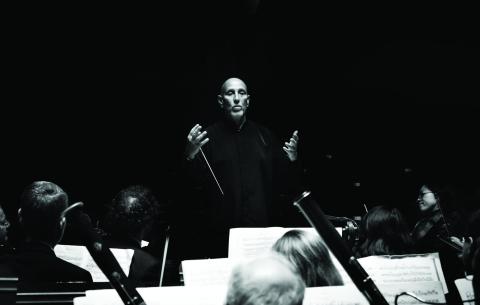This is a high-contrast black-and-white photograph capturing a dramatic scene of an orchestra conductor in action. The bald maestro, dressed in black, is the focal point as he stands against a stark black background that obscures much of his clothing, making only his head and hands visible. His right hand holds a downward-pointing baton, while his left hand is extended, as if signaling to the orchestra. His facial features appear sallow, and he looks down intently at the musicians.

The image is taken from the perspective of someone at the back or in the middle of the orchestra, showcasing the backs of several orchestra members' heads. These musicians, who include men and women with various hair colors, are seated in front of their music stands with sheet music laid out. The raised instruments visible, particularly clarinets and possibly oboes or bassoons, suggest that the woodwind section is prominently featured in this photograph. The dark background and the musicians' attire make it challenging to distinguish finer details, but the intensity and focus of the moment are palpable.